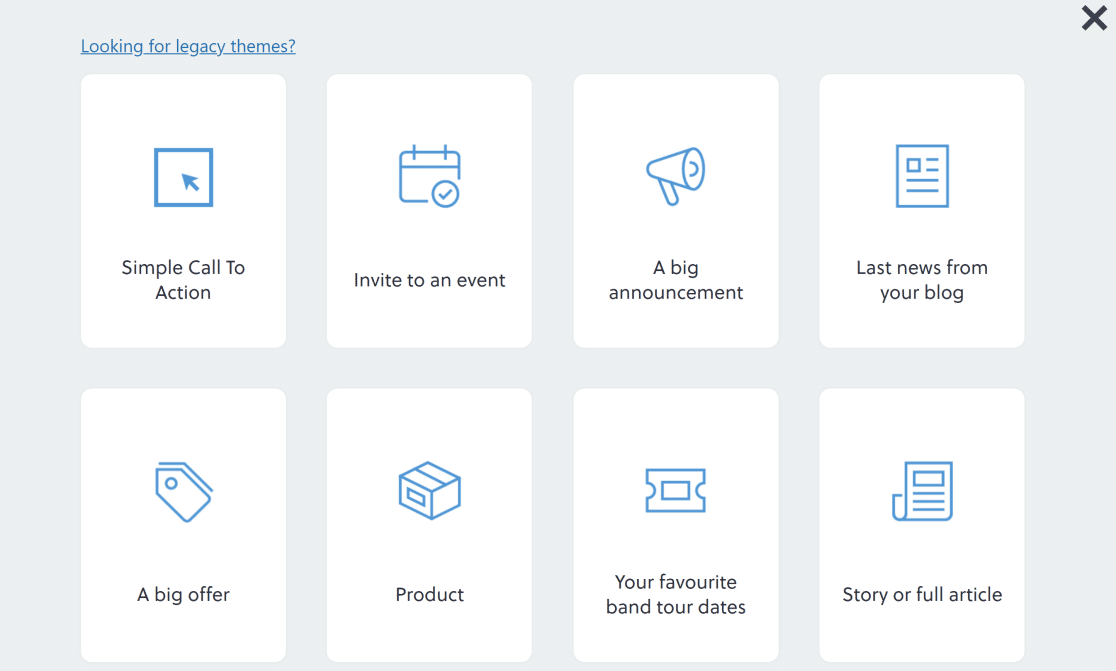**Detailed Caption:**

The image features a webpage with a gray background and various interactive elements. At the top of the page, the header reads "Looking for Legacy Themes" in blue text, positioned adjacent to a gray "X" on the far right, presumably for closing the notification or section.

The layout displays several white boxes, each containing an icon and a descriptive text:

1. **Simple Call to Action**: This section includes a blue arrow inside a square box.
2. **Invite to an Event**: Illustrated by a calendar with a check mark.
3. **A Big Announcement**: Represented by a blue megaphone.
4. **Latest News from Your Blog**: Visualized with an image of a piece of paper containing writing.
5. **A Big Offer**: Identified by a blue sale tag.
6. **Product**: Marked with a blue box icon.
7. **Your Favorite Band Tour Dates**: Symbolized by a blue and white ticket stub.
8. **Story or Full Article**: Depicted by a partially folded blue piece of paper with lines on it.

Each white box prominently features black text at the bottom, providing a summary of the function or action that clicking on the corresponding button would perform. The harmonious use of blue icons and black text against the white boxes creates a clean and visually appealing design.